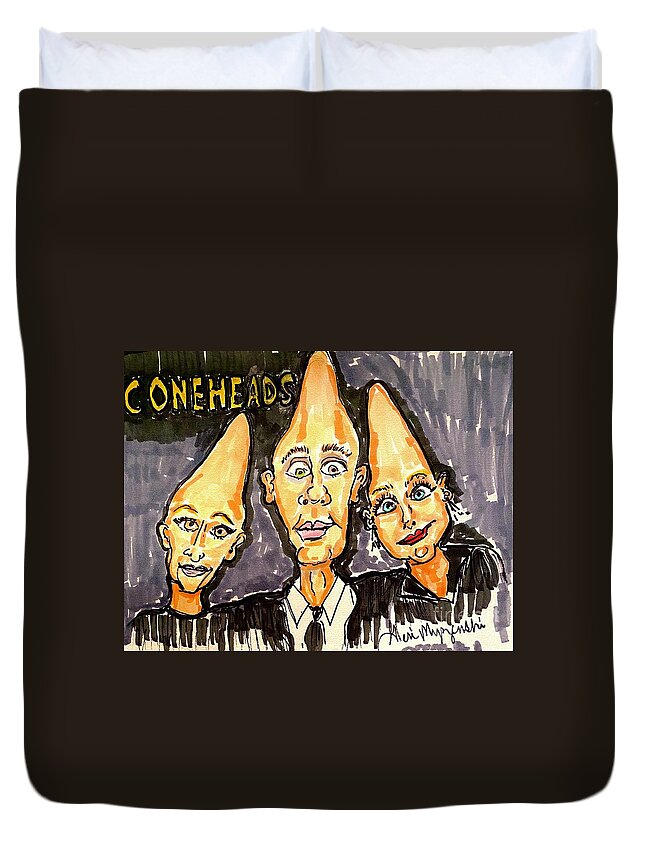This image features a detailed color marker rendering of the Coneheads, a popular skit from Saturday Night Live. The drawing is placed on a black blanket with two white pillows visible at the top, positioned on a vertically oriented bed. In the center of the image are three characters: a man in the middle, flanked by a woman on each side. All three have prominent, flesh-colored cone-shaped heads and are smiling directly at the viewer.

The man is dressed in a white collared shirt with a black tie, while the women on either side of him wear black tops with distinct black and white detailing. The background of the drawing features shades of gray with black and white painted lines, adding depth to the scene. In the top left corner of the image, there's a blackened area with gold writing that spells out "Coneheads." The style blends cartoonish elements with realism, providing a vivid yet artistic portrayal of the characters. A handwritten signature is noticeable in the bottom right corner, though it is too unclear to be legible. This detailed rendering effectively captures the whimsical essence of the Coneheads against a contrasting black and gray backdrop.